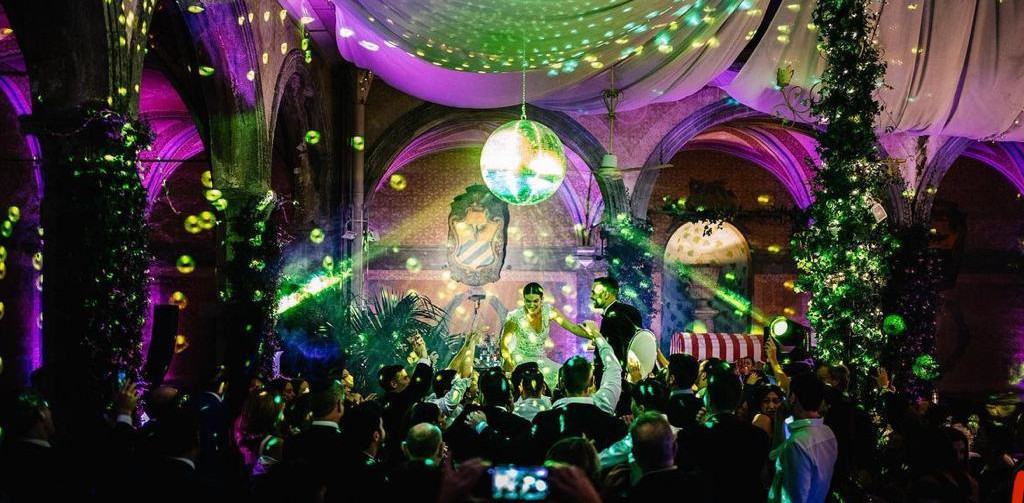The image captures an ornate wedding reception at night, bathed in vibrant purple and green lighting that illuminates the arched walls and tall trees surrounding the venue. In the center, a bride in a classic white dress and veil, and a groom in a black jacket, are lifted on white chairs by guests. Above them, a glittering disco ball casts colorful, twinkling reflections across the room, adding to the festive atmosphere. The dance floor is crowded with guests watching the couple, framed by beautifully decorated columns adorned with white flowers and lights. The ambiance, reminiscent of a classic movie scene, is further accentuated by a live performance on stage, featuring a singer dressed like Elvis, accompanied by musicians, including a drummer.